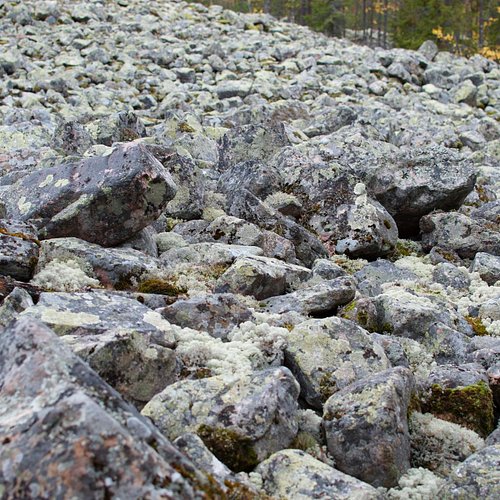This square-format color photograph depicts a field of diverse rock formations set against a backdrop of tall, green-leaved trees, suggesting a mountainside or a wooded area. The rocks, varying in size and shape, predominantly exhibit a gray and black speckled appearance with occasional brown spots. Some rocks feature whitish blotches and patches of green moss or lichen, enhancing their textured surface. The field of boulders extends across the entire frame, resembling a vast, rugged carpet of stones, possibly indicative of a lava field given its abrupt transition to dense forest along its edges. This natural mosaic creates a striking contrast between the rocky expanse and the lush greenery, lending a dynamic and compelling visual narrative to the scene.